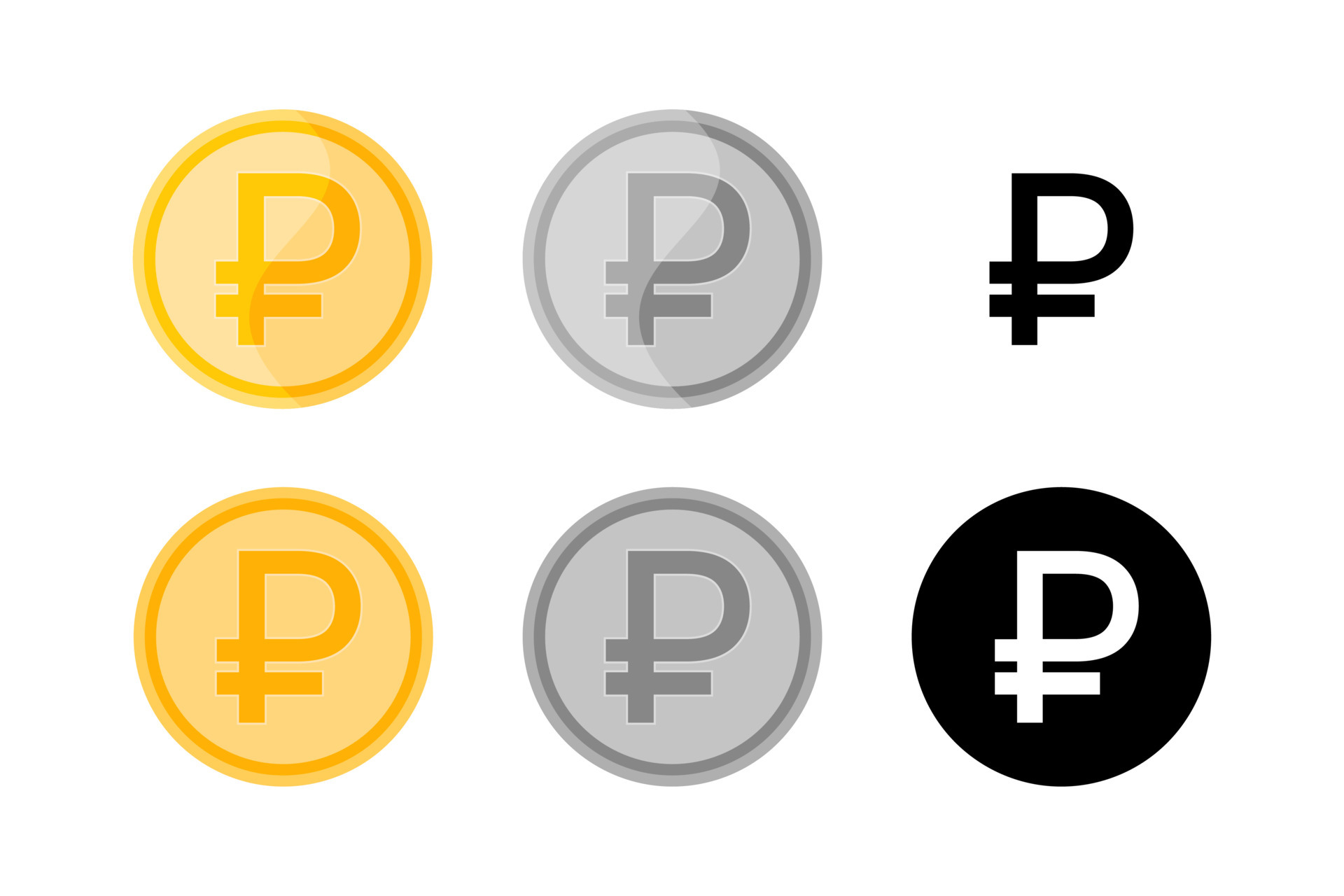The image features six circular emblems arranged in two rows of three, set against a solid white background. Each emblem displays a "P"-shaped logo combined with a cross-like extension at the base, reminiscent of a key. The emblems differ in color and background pattern, yet share similarities in their design layout. 

- The top left and bottom left emblems are predominantly gold. The top left emblem has a swirling gold gradient background, while the bottom left is a solid gold. Both have a darker gold border encasing the circular emblem.
- The top middle and bottom middle emblems follow a similar pattern but are colored in shades of gray. The top middle shows a swirling gray gradient, and the bottom middle features a solid gray background enclosed by a darker gray border.
- On the right side, the top right emblem is unique, displaying a plain black "P" symbol without any enclosing circle. Directly below, the bottom right emblem mirrors this "P" symbol in white, encompassed by a solid black circular border.